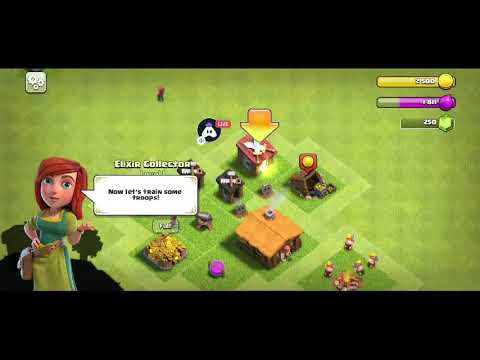The image is a screenshot of a strategy video game. The camera is pointed down at a village area built on square tiles, surrounded by a green checkered pattern of darker and lighter green grass. In the bottom left corner, there's a cartoon female character with red hair parted to the left, wearing a green dress with a light green apron. Her hair reaches down to her shoulders, and she has large eyes. One of her hands is raised to shoulder level with her palm up, while the other is on her waist, with a bag hanging across her waist down to the side of her left leg. A speech bubble next to her head, with a white background and black text, reads, "Now let's train some troops," and above it, in white text, it says, "Elixir Collection."

In the center of the image is a house with a light brown sloped roof and a gray chimney emitting smoke. Above it, a gold-colored arrow points straight down at another building. Several buildings are arranged in a checkered pattern across the village. The bottom part of the screen features green checkered tile patterns. In the upper right corner, there are three horizontal resource bars colored orange, purple, and dark green. In the upper left corner, there's a gray icon with white gear symbols, indicating settings. The entire image is dominated by these elements, typical of a mobile game interface.